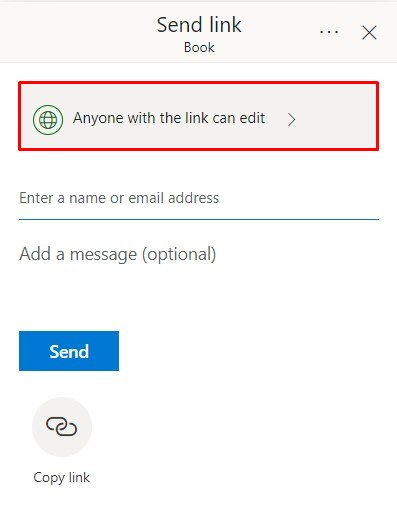The image depicts a user interface, likely from a mobile app or a desktop application, designed for sharing content. The top section features a "Send Link" title along with three vertical dots, suggesting more options, and an "X" button to close the window. Below this, the word "book" appears in gray text.

Highlighted within a red rectangular border, there is a message stating, "Anyone with the link can edit," accompanied by a small green globe icon just before the text. A forward arrow follows, indicating continuation of the process.

Moving further, there is a blue-underlined field labelled "Enter a name or email address," which is currently blank. Below this, a section marked "Add a message" is encased in quotations, denoting that this step is optional.  

At the bottom, a prominent blue "Send" button with white text stands out. Adjacent to this, a "Copy Link" option is represented by a chain link icon, symbolizing the function to duplicate the sharing link.

The entire interface appears on a clean white background, devoid of any branding, logos, or advertisements, suggesting that it might be a simplified or cropped view of a larger application.